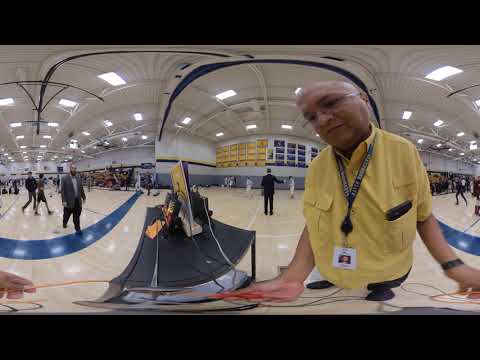This distorted and peculiar 360-degree photograph taken in a gymnasium prominently features a man on the right side of the image. He appears to work there, as evidenced by the black lanyard with an ID tag hanging around his neck. The man is wearing a yellow button-up shirt with a smartphone or similar device in his pocket, glasses, a watch, and is bald with lighter skin. The gymnasium space can be seen behind him, showcasing light tan, glossy wooden floors marked with white stripes. The gymnasium's ceiling is supported by steel girders and equipped with fluorescent lights. On the walls are purple and yellow banners alongside a series of plaques. Various athletes dressed in white martial arts uniforms and a few men in suits can be observed walking around the space. A black table with computer equipment is also visible, as well as what appears to be a ramp or bench with a brochure and possibly an ice skate on top. The image combines several elements, including a basketball court with a blue trim and gray and white walls, contributing to the warped, magnifying glass effect that distorts the entire scene.